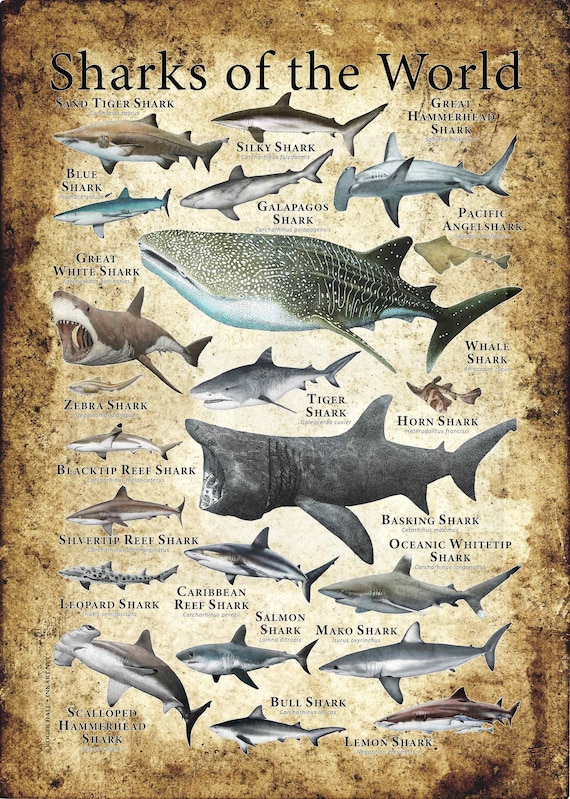The vertically oriented poster, titled "Sharks of the World" in bold black text at the top, showcases an array of approximately 20 different shark species against a textured, tan background that transitions from a lighter beige in the center to a darker, almost burnt-looking brown around the edges. Central to the poster are two prominently featured sharks: a large Whale Shark displaying a distinctive greenish top with white spots and a white belly, and beneath it, a massively open-mouthed Basking Shark in dark gray. To the left of the Whale Shark is a smaller Great White Shark, recognizable by its gray and white markings. Scattered across the poster are various other sharks, each labeled with their names, such as the Great Hammerhead Shark on the right with its distinctive hammer-shaped head, and the Blue Shark to the left noted for its blue body. Other notable species include the Tiger Shark with its striped body, the swift Mako Shark, the spotted Leopard Shark, and the flat-bodied Angel Shark that vaguely resembles a stingray. The rough, ripped appearance of the background with hints of blackness through the "holes" adds an aged, maritime feel, enhancing the visual context of these diverse marine predators.